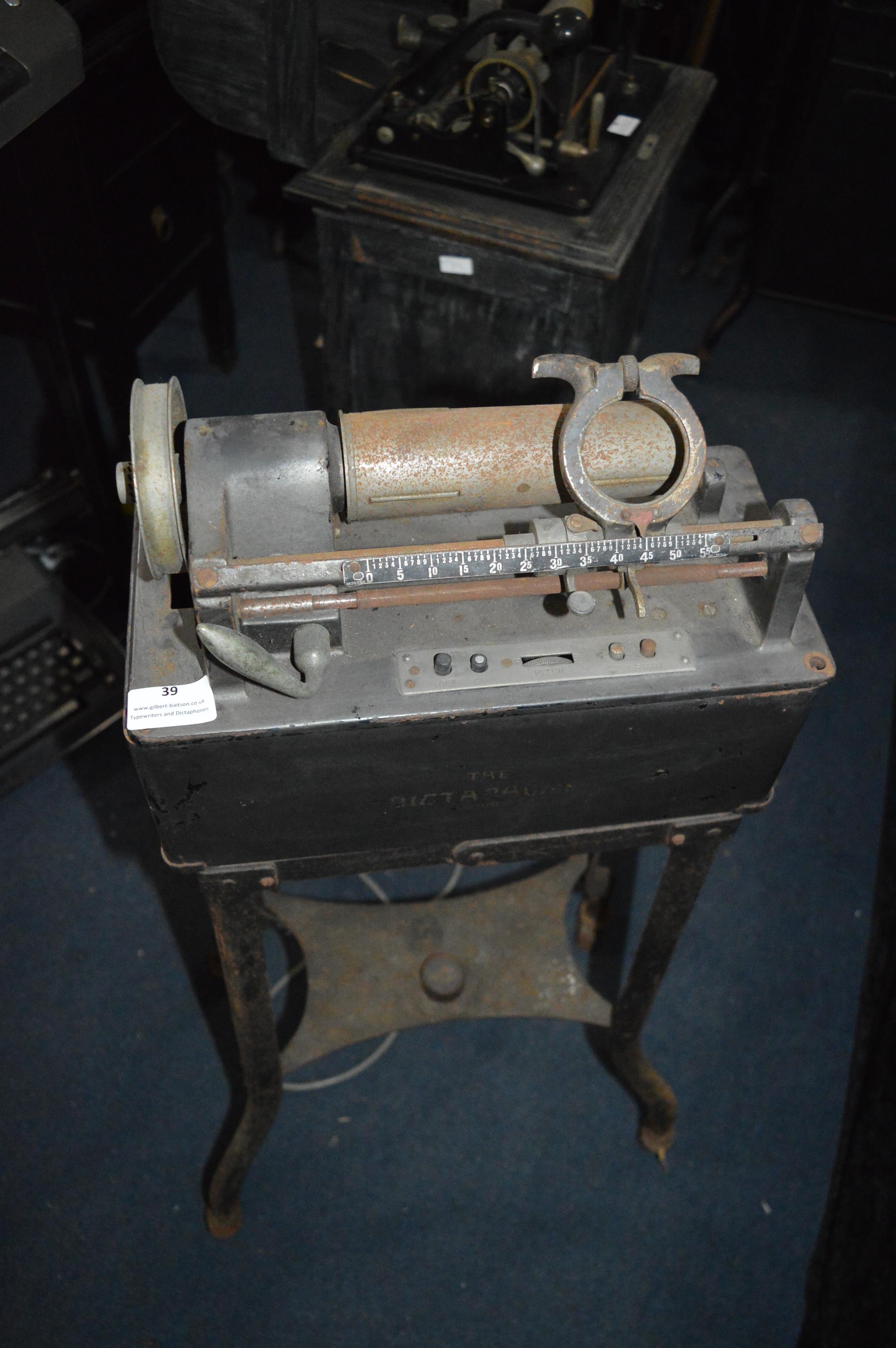The image features an old, worn-out mechanical device that stands on a dated blue carpet. The machine appears rusty and aged, with various areas showing significant wear. It is predominantly metal and integrated into or placed upon a wooden table with wooden legs, giving the impression that it's been out of use for some time. The machine is equipped with several cylinders on top, a silver ruler for measuring on the front, and a dial that can be adjusted. A notable feature is a white sticker with the number "39" in black text attached to the left side of the machine, further indicating its antiquity.

Despite its potential confusion with a sewing machine or weight scale, the missing elements like a stepping plate or sewing needle direct attention to its ambiguity. The device has multiple knobs on a front plate, possibly suggesting an old industrial purpose. In the background, there are various vintage machines and a typewriter, contributing to the overall dusty and dimly lit environment. The image is illuminated by a flash, highlighting the machine against the darker backdrop.